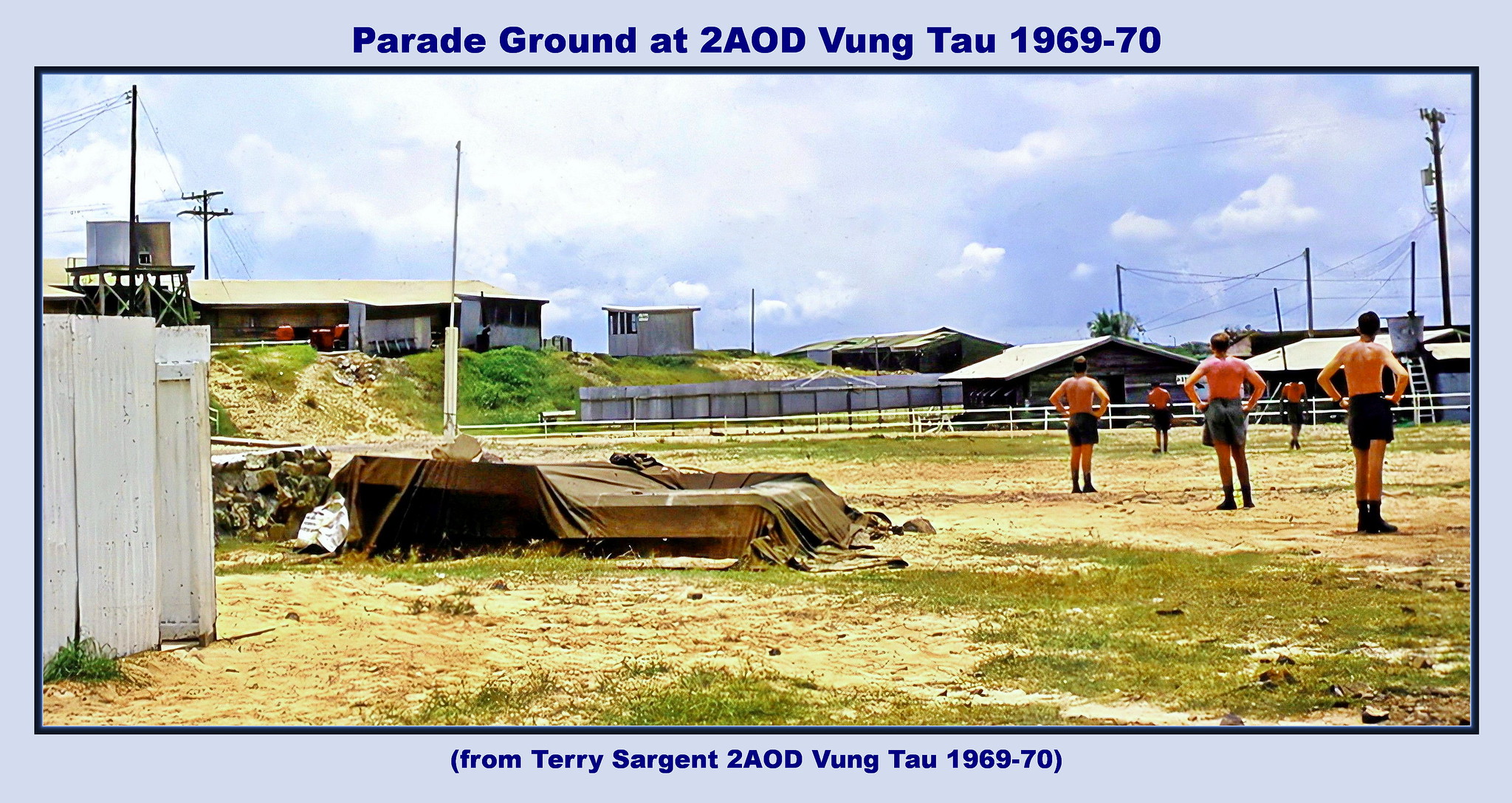In the photograph titled "Parade Ground at 2AOD Vung Tau 1969-70" (courtesy of Terry Sergeant 2AOD Vung Tau 1969-70) and bordered by light blue text, five men stand on a patchy, dead grass field littered with wood, metal debris, and trash in the foreground. The men, situated on the right side, wear only shorts, socks, and shoes with their hands on their waists, gazing into the distance. Above them, a very blue sky, thick with clouds, stretches wide. In the background, a fence runs parallel to several shed-like and metal-clad work buildings, set against the landscape likely indicative of a military base. Visible power lines and distant shacks underscore the utilitarian environment.